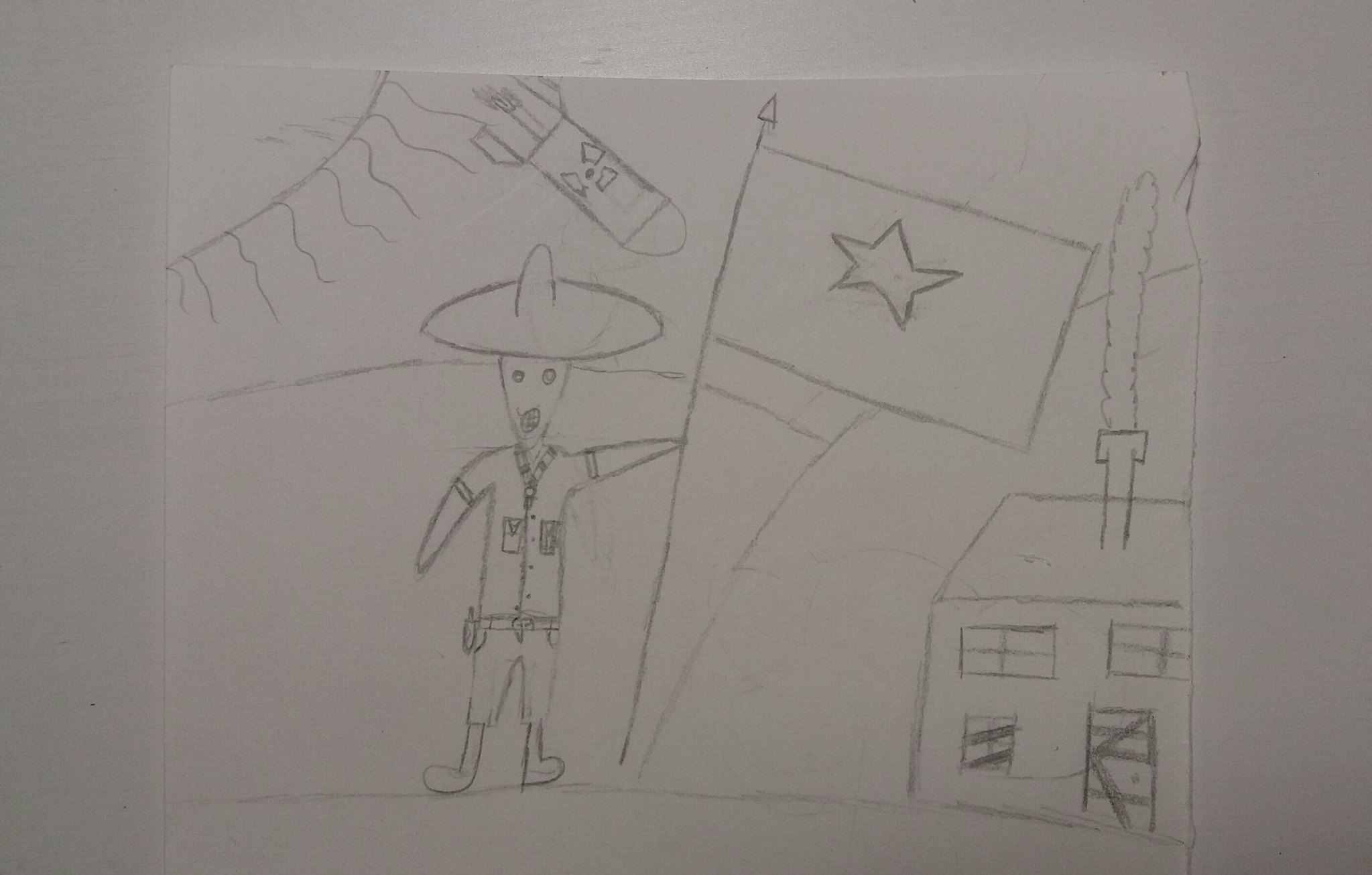The image showcases a detailed, pencil-drawn scene that appears to be a child's imaginative rendering. Central to the composition is a figure, possibly a cowboy or sheriff, characterized by a triangular head, round eyes, a mouth, flipper-like arms, and club feet. The figure, outfitted in a sombrero, a short-sleeved shirt with pockets, and shorts, stands firmly holding a flag with a five-pointed star. To the right of the figure is a small cabin featuring a central chimney emitting a cloud-like plume of smoke, indicating warmth within. The cabin has two upper story windows and additional windows and a door on the first floor. Above the scene, a quarter-circle sun with linear rays occupies the upper left corner, while a missile — with a somewhat ambiguous, face-like design — appears to be hurtling toward the flag. The entire drawing is set against a clean, white background, emphasizing its playful, sketch-like charm.